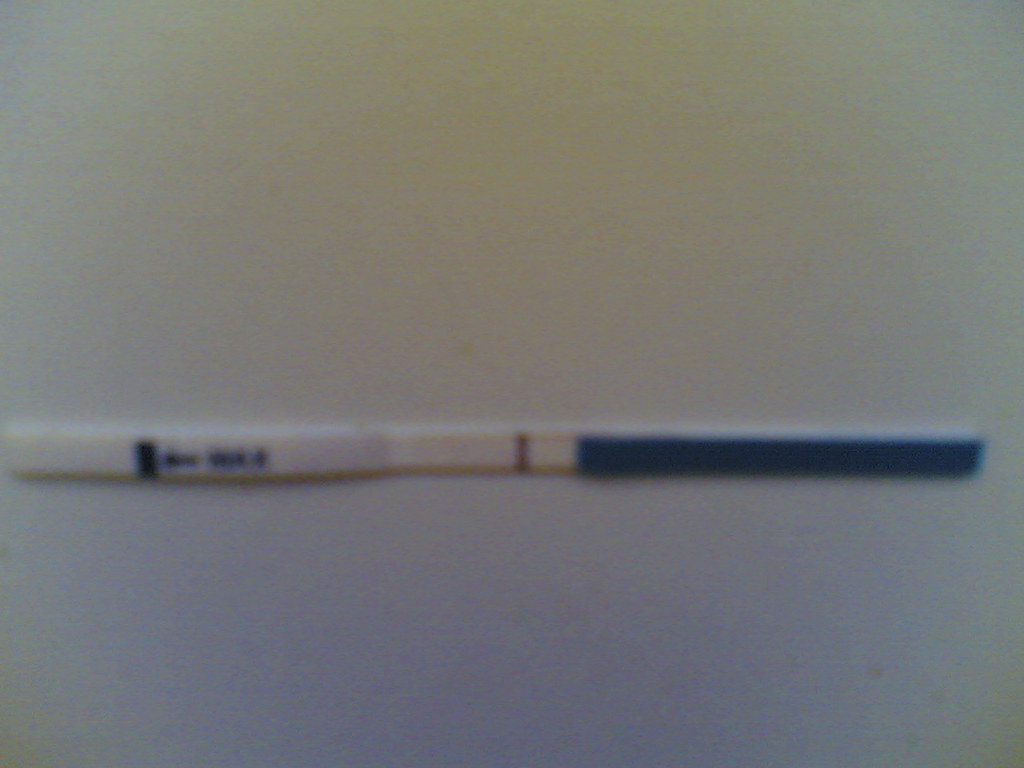A very blurry photograph captures an unidentified object against a variegated gray background. The object, which is horizontal, appears elongated and narrow. Approximately one-third of it is blue, likely constituting a handle. The remaining two-thirds are white and feature a thin red stripe, along with some indiscernible dark blue writing and a short dark blue line. Due to the image's lack of focus, the text remains unreadable. Both terminations of the object are blunt, with one end white and the other blue, and there is no discernible tool or attachment at the white end, making it challenging to ascertain the object's true nature.